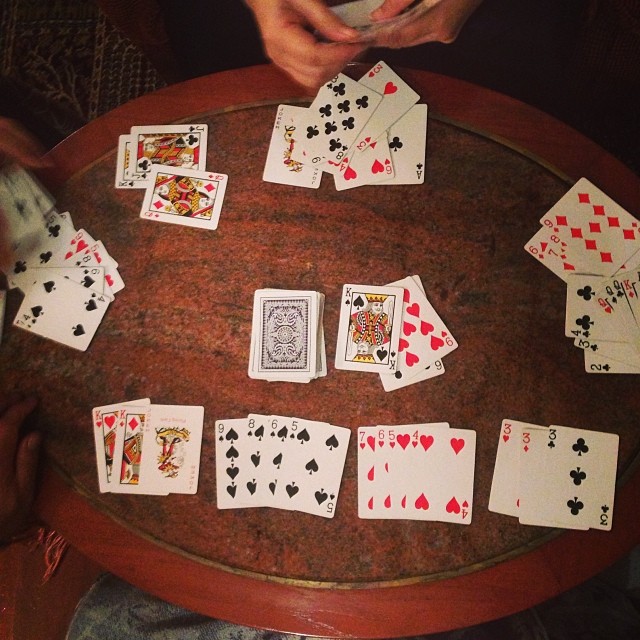In this image, we see a group of two, possibly three people engaged in a game of cards. Featured prominently at the top of the image are hands holding a pair of white cards. The table beneath them has a rich dark red border, transitioning to a darker brownish hue with gray lines intersecting in the middle. The cards themselves have distinctive designs, showcasing a white background with intricate gray and blue half-circle swirls.

Scattered across the table are various playing cards: a king of spades is positioned near the top, along with a nine of hearts and a six of spades. In the top left corner, a queen of diamonds, a jack of clubs, and a king of hearts are visible. Additionally, a joker card lies on the left side, partially covering a king of diamonds and a king of hearts. The assortment of colors and numbers on the cards adds a dynamic and vivid touch to the scene of this card game.